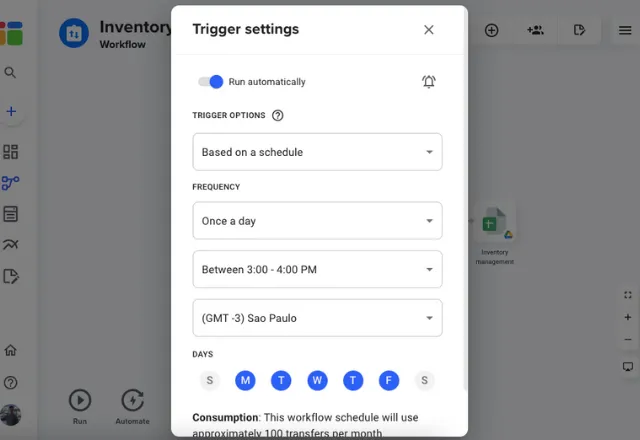The image is a screenshot of a computer interface displayed against a darker gray opaque background. On the left-hand side, there is a vertical navigation column with icons. The topmost label in this column reads "Inventory" in black text, followed directly underneath by "Workflow." 

The interface features multiple elements, including a blue circle icon and a suitcase-like icon with more blue imagery. A prominent pop-up box in the center is titled "Trigger Settings" with a close (X) button at the top. Within this pop-up, there is an enabled slider next to the label "Run Automatically." Next to the slider, there is a bell icon that visually indicates the feature is active.

Below the slider, a section labeled "Trigger Options" features a question mark icon inside a circle. A checkbox option labeled "Based on a Schedule" follows, highlighted by a lighter gray background. Additional settings specify the trigger schedule: a frequency set to "Once a Day," with a selectable time range dropdown currently showing "3:00 PM - 4:00 PM." The time zone is set to "GMT-3:00 São Paulo," also adjustable via a dropdown menu.

A weekly schedule displays days of the week, each accompanied by small circles underneath. Sunday and Saturday have gray circles, while Monday through Friday have blue circles, indicating active days for the triggered event. There is an information section stating that the workflow schedule will use approximately "100 transfers per month," described under the heading "Consumption." 

Overall, this interface visually presents a detailed workflow schedule configuration and its associated settings.